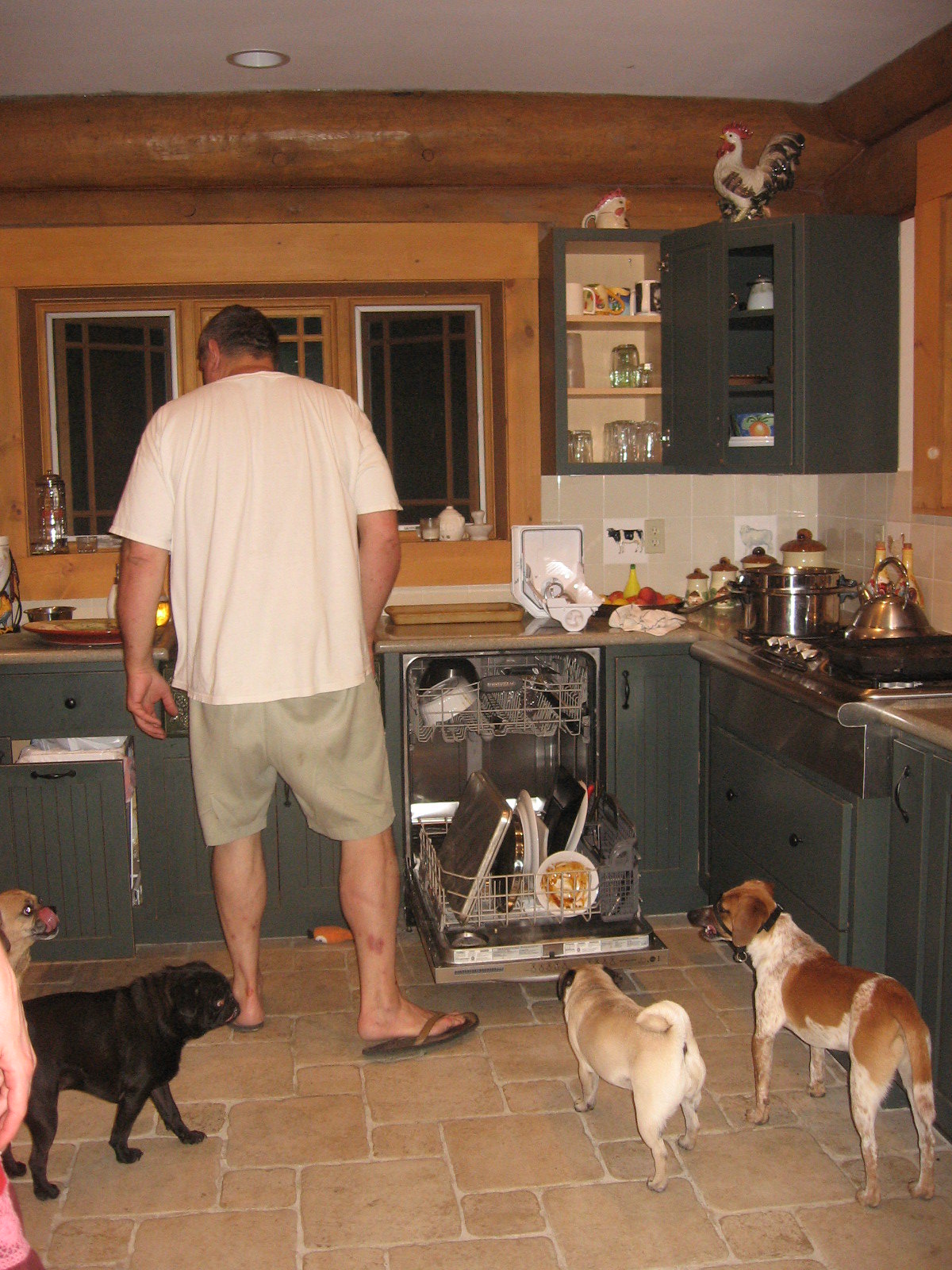This photo captures a slightly dated kitchen that seems to be from around 15 to 20 years ago. The kitchen features stone-look tile flooring and gray, old-fashioned cabinets that evoke the style of the 60s or 70s. The countertop appears to be brown marble, with an open dishwasher revealing the lower rack filled with pots, pans, and a circular saucer. Above the sink, there are three windows that let in natural light, reflecting off wood-grain walls and a wooden ceiling with inset lighting. 

The focal point of the image is a man standing near the open dishwasher. He is dressed in a white t-shirt, light green or khaki shorts, and brown flip-flops, with his back turned to the camera. He's a tall, large man with notably developed calves, seemingly engrossed in a task on the counter.

Four mid-sized dogs are gathered around him, all attentively watching his actions. The dogs vary in color; one is black, another is sable, a third is brown and white, and the fourth, a beige dog, has its tongue out, licking its nose. In the background, a hint of another person is visible, with only a hand showing on the left side of the photograph. The busy countertop also holds some appliances and jars of flour and sugar, adding to the everyday, lived-in feel of the scene.